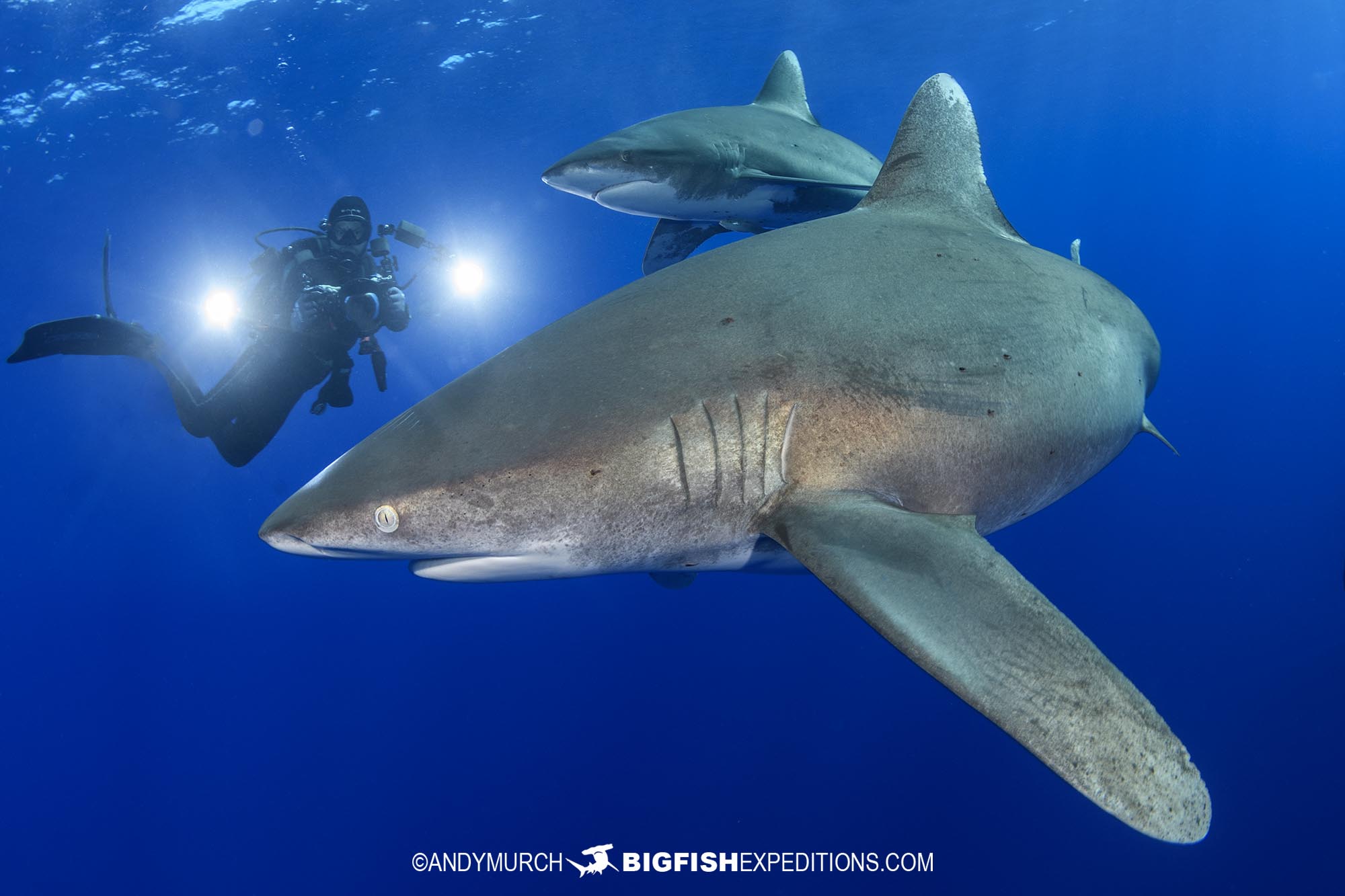This captivating underwater photograph captures two majestic sharks swimming in the deep blue ocean. The sharks are dark gray with stark white undersides, and their beady, white eyes stand out against their sleek bodies. One shark, slightly sideways with its mouth slightly open revealing no teeth, dominates the foreground. Its fins and gills are clearly visible. Just behind this shark, another one appears to be circling around, slightly higher and to the left. The secondary shark features a hint of light brown along its side.

To the left of the composition, a scuba diver clad in black diving gear is keenly focused on capturing the marine scene. He wields a large camera in his hands while carrying two additional large white cameras mounted near his shoulder pads. He is equipped with large flippers on his feet, and bubbles can be seen rising to the water's surface above him. Faint reflections of stars from the dark surface add a magical touch to the scene. The diver's lights cast a gentle illumination on the sharks, highlighting their features against the deep blue background.

At the bottom center of the photograph, a watermark displays a copyright symbol followed by "Andy Murch" in white text. Below it, a small image of a hammerhead shark appears alongside the text "BIGFISHEXPEDITIONS.COM," all in uppercase white letters. This well-composed image beautifully captures the serene yet powerful essence of these oceanic predators and their environment.